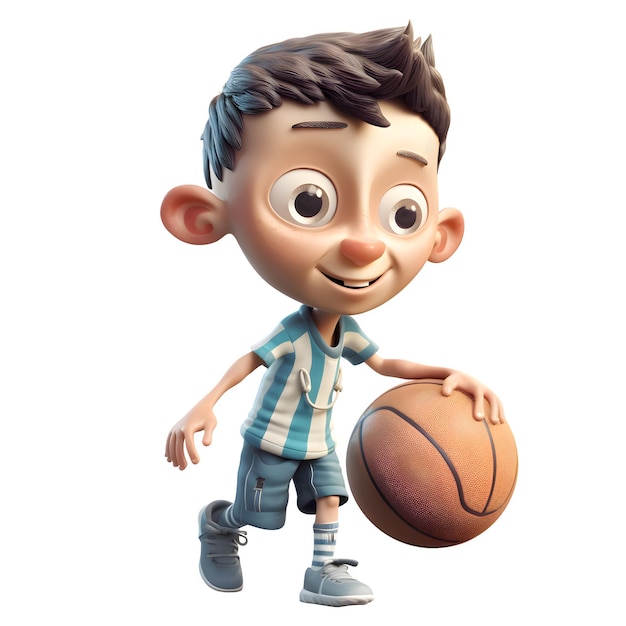This is a highly detailed, animated Pixar-style image of a boy with notable features and a vivid personality. The boy has an exaggerated, cartoonish appearance, characterized by his large, round ears that protrude prominently from the sides of his head. His short, brunette hair is styled in a spiky manner, some of which sticks up. His smiling face is adorned with gray eyes, a pair of prominent front teeth, and a notably red, rosy nose. He exudes a happy expression, complete with a raised eyebrow. He wears a vertically striped t-shirt in light blue and white, complemented by baby blue shorts. His blue and white horizontally striped socks peek out from gray sneakers. The image shows him in motion, dribbling a basketball almost as big as his head. The background is a plain white, enhancing the focus on the boy, indicating that this might be a character design concept. There is no text present in the image.